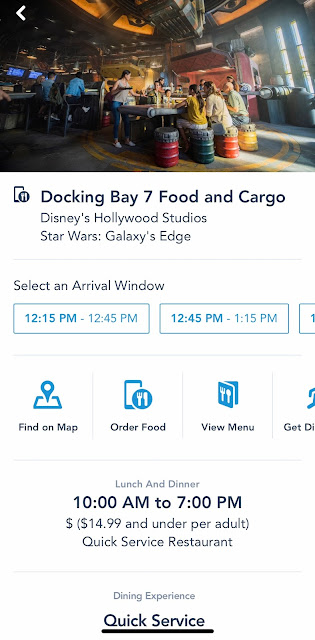**Caption:**

A screenshot of a food application on a smartphone captures the interface for Docking Bay 7 Food and Cargo, a Star Wars-themed restaurant located in Disney's Hollywood Studios, Galaxy's Edge. The hero image at the top depicts a vibrant, immersive setting where guests sit on metal drums in a pirate or Star Wars-inspired ambiance. People are seen milling around, enjoying their food in this stylized establishment.
 
Below the image, a smartphone icon with a knife and fork inside a circle is placed on the bottom right. The text next to it reads: "Docking Base 7 Food and Cargo, Disney's Hollywood Studios, Star Wars: Galaxy's Edge." 

Below this section, options for selecting an arrival window are presented, including 12:15 PM to 12:45 PM, 12:45 PM to 1:15 PM, and another partially hidden option in blue text, enclosed by a thin blue line. 

Further down, a row of icons offers additional functionalities: a map pointer labeled "Find a Map," another knife and fork icon with "Order Food," an open menu icon indicating "View Menu," and a partially visible "Get Directions" icon cut off at "DI."

Centered and in light gray text, it reads "Lunch and Dinner," followed by bold black text displaying the hours of operation: 10 AM to 7 PM. At the bottom, a price range indicates "$14.99 and under per adult," highlighting it as a quick-service dining experience.